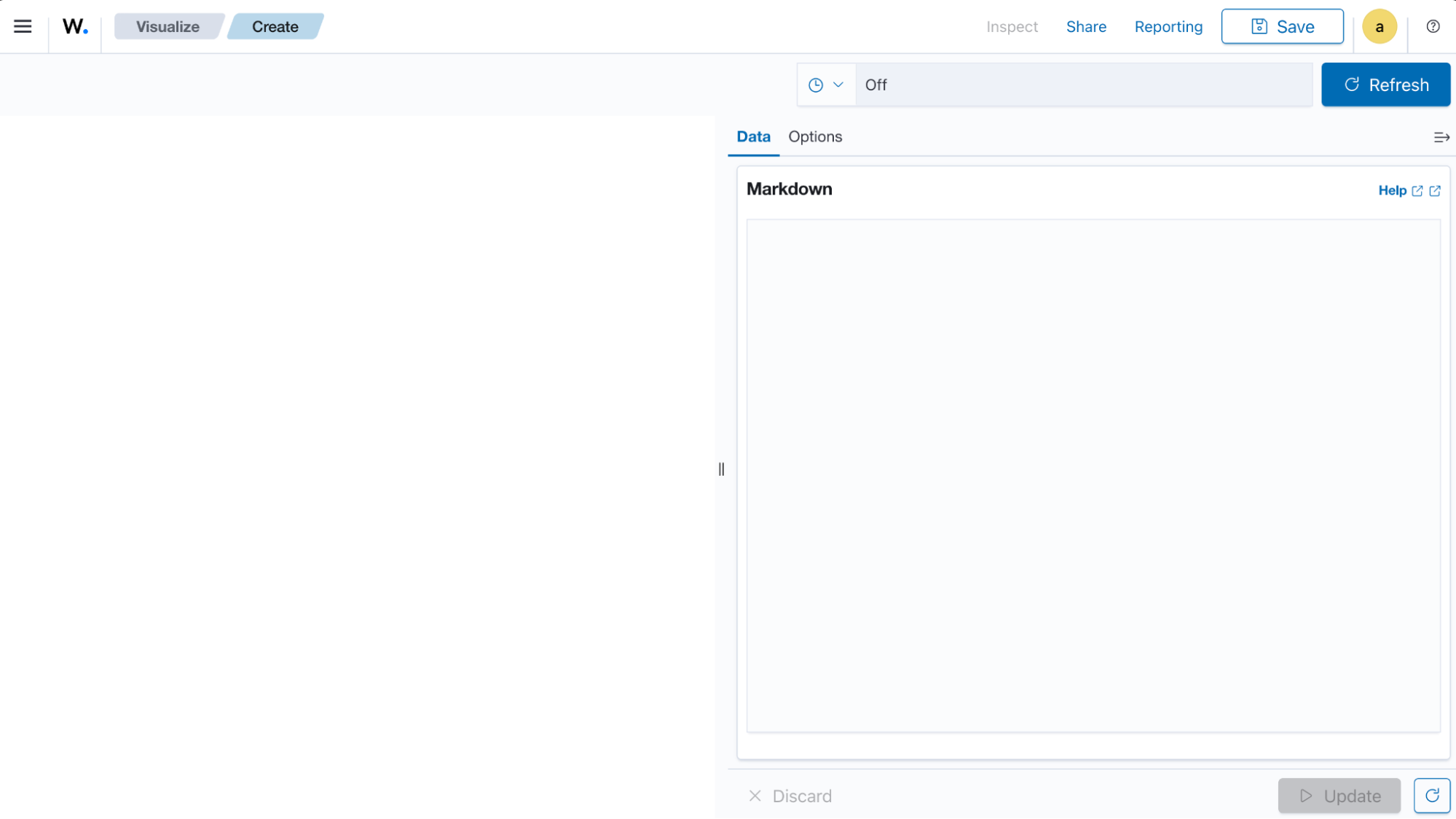The image displays a screenshot of a website, divided into what appears to be two main sections. At the top left corner, there is a prominent black "W" accompanied by three horizontal black lines, which might be indicative of a menu. Adjacent to this are two clickable elements: "Visualize" within a gray parallelogram, and "Create" housed in a blue parallelogram.

Continuing towards the right, the words "Inspect," "Share," and "Reporting" become visible—though "Inspect" appears faint and less noticeable. In contrast, "Share" and "Reporting" stand out in a blue font. Further right, the word "Save" is displayed, and nearby, a letter "A" is encased within a yellow circle.

There is a blue refresh button, labeled "Refresh" in white, and an option indicating "Off" in the clock section. The dropdown menu reveals a blue-highlighted "Data" link with an underline, alongside "Options" and "Markdown" in black print beneath. Additionally, there is a help section, and towards the bottom, an "X" labeled "Discard." An update arrow and another refresh button are present at the bottom right corner.